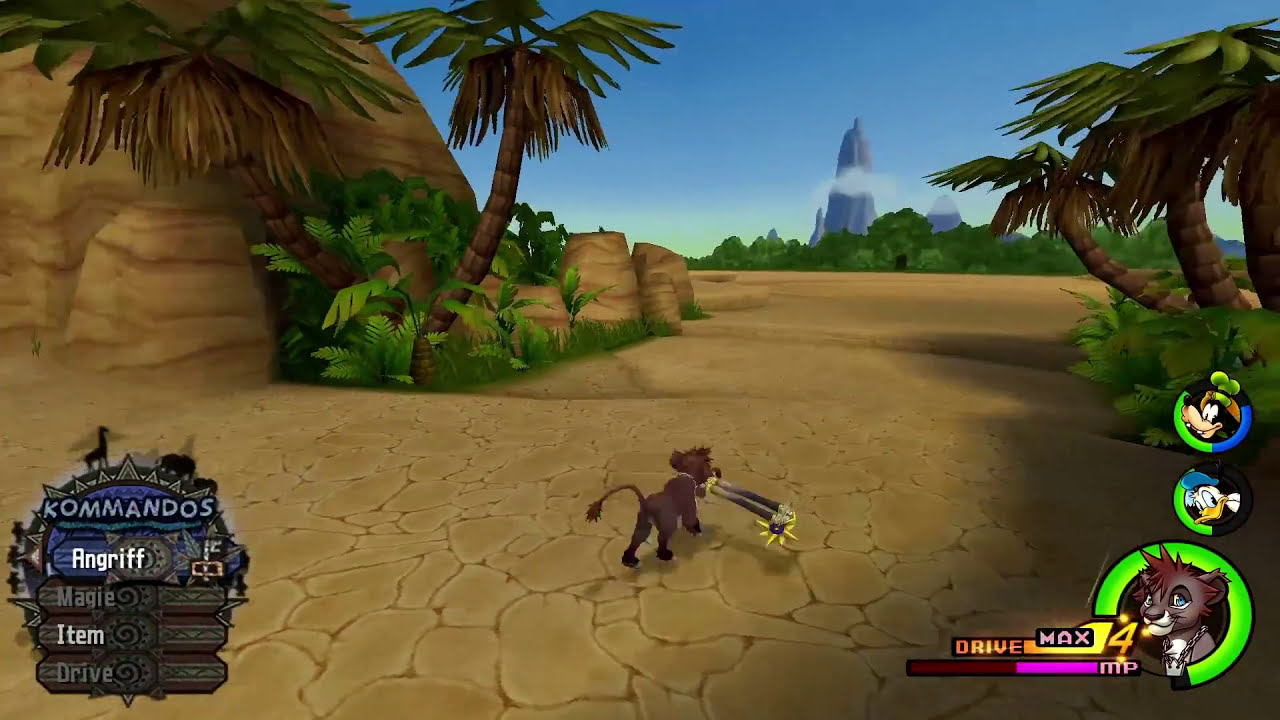The screenshot depicts a vivid scene from a video game with a prominent outdoor landscape featuring sandy, flat, stone-like ground. In the foreground, a brown lion cub is visible, carrying a spiked ball weapon in its mouth. The terrain includes a large grassy plain intermingled with a stony area and a dessert-like expanse, bordered with palm trees and green shrubs. In the distance, a distinctive mountain peak rises sharply against a bright blue sky with a tree line indicating a heavily forested area. On the lower left corner, the interface displays the label "Commandos" (with a K) and an array of score items including "Angriff Maggie," beneath a circular and rectangular blue and brown design. The bottom right of the screen reveals more score details: various icons and a red and pink bar labeled "drive max for MP." The icons include familiar figures resembling Donald Duck, Goofy, and a spiky-haired lion, encased in green-bordered semicircles.